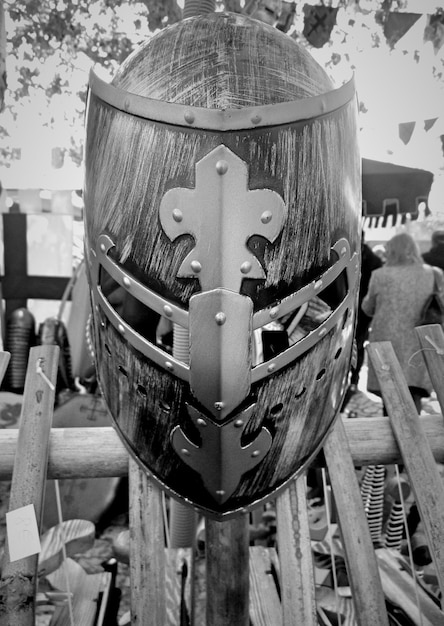This black-and-white photograph features a close-up of a knight's helmet displayed on a wooden rack, likely imitating medieval design. The helmet, which appears large due to the closeness of the shot, is the focal point of the image. It has a rounded top and a shield-like visor that can be lifted to reveal the face, complete with rectangular eye slits reinforced with rivets. The nose guard is a prominent, strong piece, and there are small ventilation holes near the mouth area. The helmet looks weathered, with visible scratches suggesting wear. Above and below the nose area, there are decorative motifs, likely fleur-de-lis. The background shows handles of swords on a rack, people walking by, and banners and flags, adding to the medieval atmosphere. Trees and a large flag with a cross are also visible, though blurred and less distinct. Overall, the image captures the knight's helmet in a detailed and atmospheric manner.